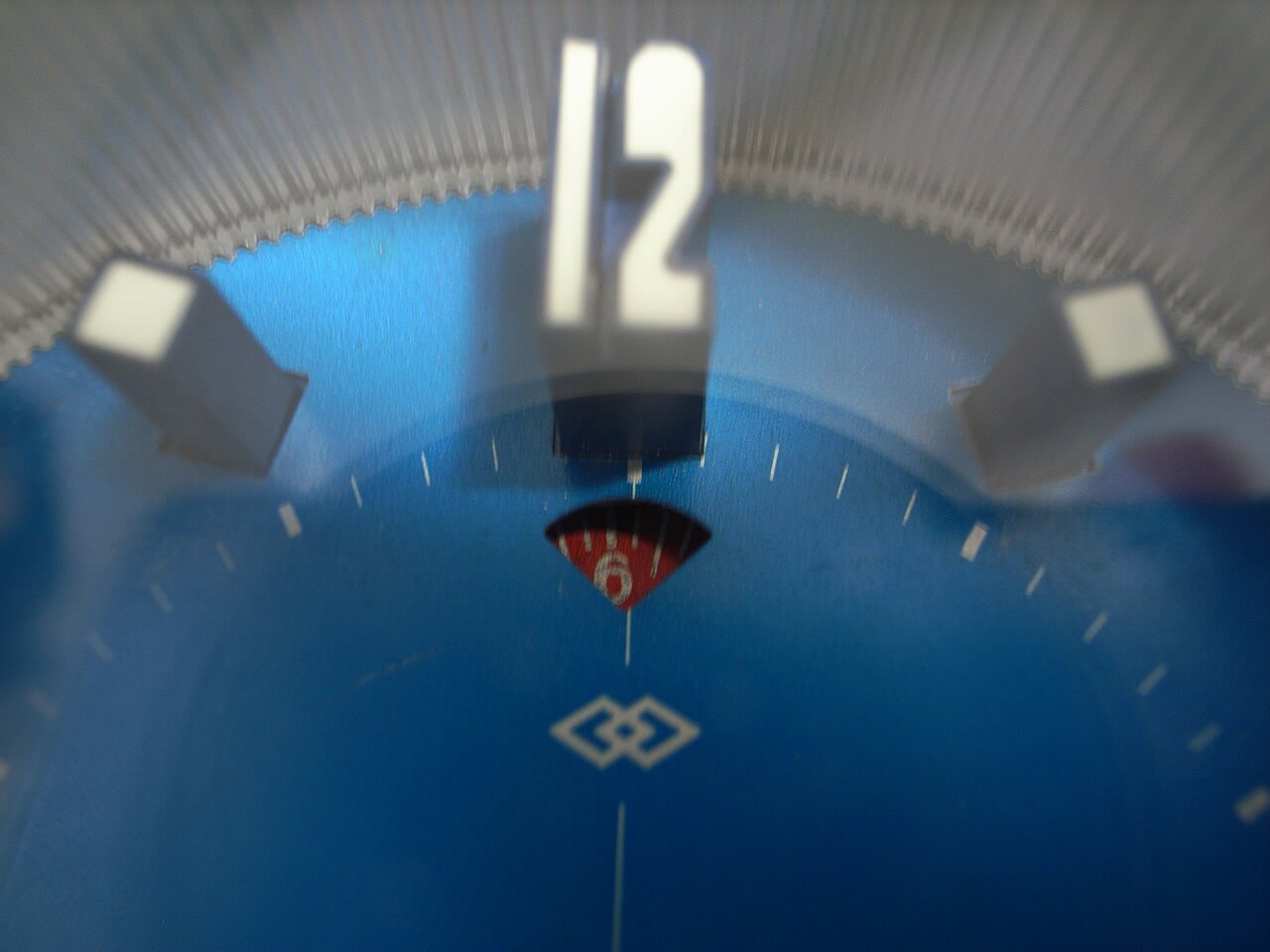This image is a detailed, close-up view of a clock face, showcasing the upper portion where the number 12 is prominently featured at the center near the top, extending outward with a metallic silver base and white top. Below the 12, recessed into the rich, dark blue clock face, is a small red wedge-shaped cutout displaying the number 6 in white, with radiating lines above it. On either side of the 12, the pegs for the numbers 11 and 1 protrude slightly, each with a black base and a white tip. The clock face itself features a series of minute markers as small dashes encircling the numbers, and is bordered by a metallic silver rim, which has slotted details. A clear, white semicircle arches above the 12, adding texture to the design. Additionally, a white line with two intersecting diamonds runs horizontally below the red 6, leading off to the right.